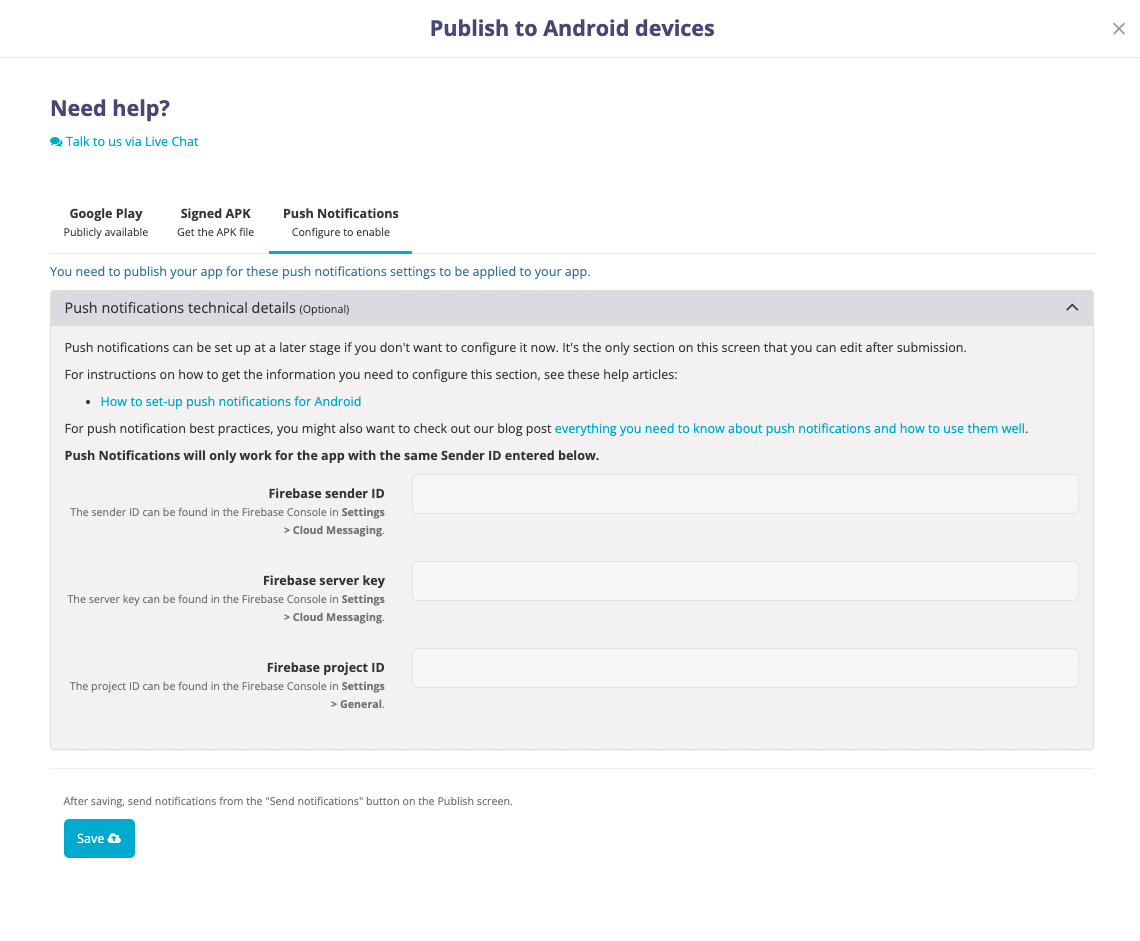The image appears to be a screenshot of a settings or configuration page for an application, tailored towards publishing and managing push notifications for Android devices. The main background is primarily white, designed for clarity and ease of reading. At the top, in dark blue text, a heading states "Published to Android Devices," accompanied by a light gray close button in the top right corner for exiting the page. Directly underneath, there's a help prompt in smaller text that says "Need help?" followed by a link in blue text suggesting "Talk to us via live chat."

The screen is divided into three main options. The leftmost option is currently selected, indicated by a blue line underneath it. This option is labeled "Google Play" and includes sub-options such as "Publicly available signed APK," "Get the APK file," and "Push notifications configured to enable." A notice below this selection warns users that they need to publish their app for these push notification settings to be applied.

A prominent gray info box occupies a central part of the screen, its header in darker gray text labeled "Push Notifications Technical Details (Optional)." The body of this box states that push notifications can be configured later and explains that this is the only section that can be edited after submission. For further instructions, users are directed to various help articles linked within the text, including "How to set up push notifications for Android" and a blog post titled "Everything You Need to Know About Push Notifications and How to Use Them Well."

Highlighted in bold text next, it states that "Push notifications will only work for the app with the same sender ID entered below." Following this are fields for the necessary push notification settings with instructions and placeholders:

1. **Firebase Sender ID:** The label informs users that this ID can be found in the Firebase console under Settings > Cloud Messaging. The corresponding input box is currently empty.
   
2. **Firebase Server Key:** Similarly, this key is to be retrieved from Firebase Console under Settings > Cloud Messaging. This input box is also empty.

3. **Firebase Project ID:** Noted that this ID can be found in Firebase Console under Settings > General, with another empty input box for user entry.

At the bottom of the form, a detailed instruction explains that after saving these settings, push notifications can be sent using the "Send Notification" button on the publish screen. Finally, a large, teal-colored button labeled "Save" in white text is placed at the bottom of the page, intended for users to save their configuration inputs.

This cohesive layout enables users to methodically configure and manage push notifications for their Android applications with reference links provided for any required guidance.